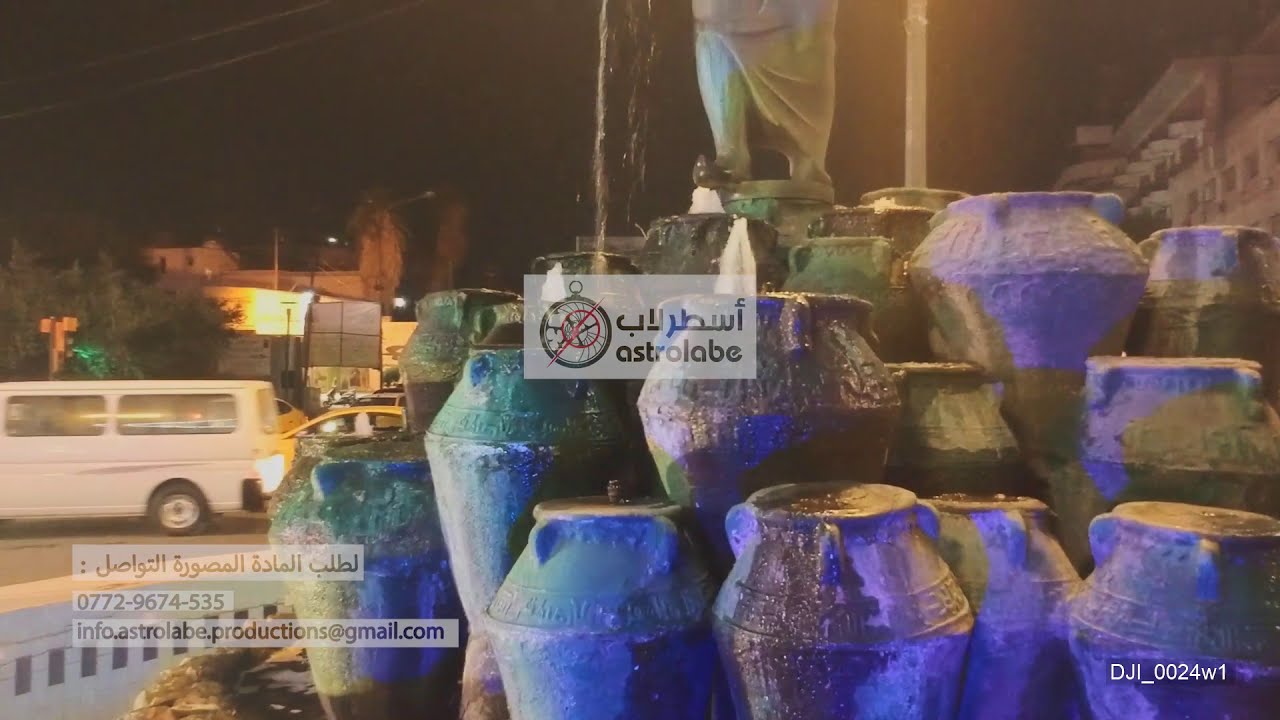The image captures an outdoor nighttime scene featuring a pyramid-like arrangement of large metal vases in blue, green, and yellow hues, structured to form a cascading fountain. The vases, made of durable material and possibly aged, flow water from one to the next, culminating at a statue above, of which only the lower half—showing legs clad in a crease-marked gown—is visible. The foreground displays personal contact details, including a phone number and an email address (info.astrolabe.productions@gmail.com).  The setting has a Middle Eastern or possibly Arabic ambiance, suggested by inscriptions and a watermark depicting a globe with a red line alongside more Arabic writing that reads "Astrolabe." To the bottom left, three transparent rectangles list further information, and a large white van is parked sideways with other vehicles and buildings in the background, all under a black night sky. In the lower right corner, text reads "DJI_0024_w1." The scene also includes streetlights and a few trees, collectively portraying a vibrant nightlife atmosphere.